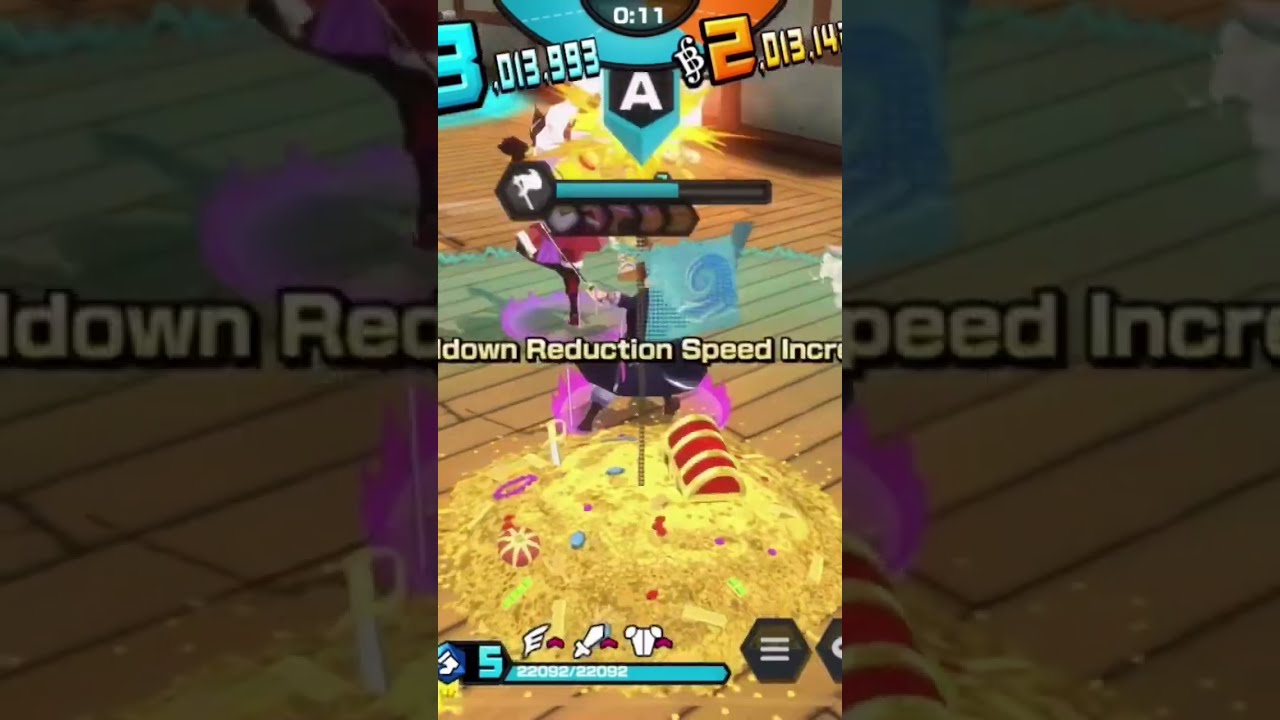The screenshot appears to be from a computer game featuring a vibrant, cartoony character positioned centrally in front of a lavish treasure hoard on a wooden floor. The treasure pile includes gold coins, multicolored jewels, and a treasure chest, with scattered swords and additional riches. The background is a golden blob behind a gray progress bar filled about two-thirds with blue, while above it is a life bar overlaying part of the character. Displaying scores and game metrics, the image includes a score of 3,000,013,993 and a countdown timer showing 11 seconds at the top. Text elements include phrases like "down reduction speed increase" and “INCR,” with numbers such as 2,292/2,292 associated with the life bar. The image appears in a three-panel format: the central panel, which is smaller, showing the main scene, and two larger zoomed-in side panels that replicate the scene with a darker tint to fit the landscape orientation.